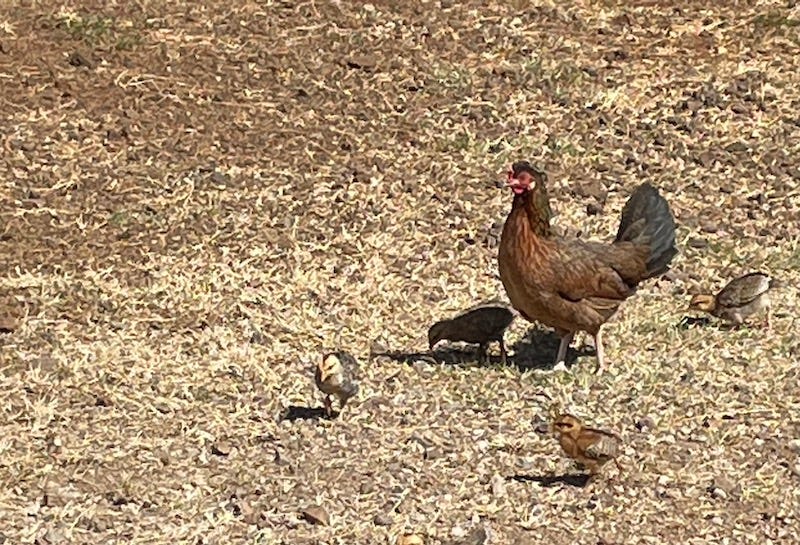In this landscape-oriented color photograph, a mother hen is captured in a dirt-filled outdoor setting speckled with yellow hay. The hen stands in profile on the right side of the image, midway up, with her beak pointing left and her black-tipped tail feathers fanned out to the right. She has a brown body, a light tan beak, red facial features, and light tan feet. Surrounding her are four baby chicks: one grey and white chick close to her, another grey chick pecking at the ground in front, a brown chick facing the viewer at the bottom left, and another brown chick standing in profile at the bottom right. The scene is free from fences or pens, focusing on the natural interaction between the hen and her chicks amidst the sparse, hay-speckled dirt. The photographic style embodies representational realism, providing a detailed and lifelike portrayal of the subjects.